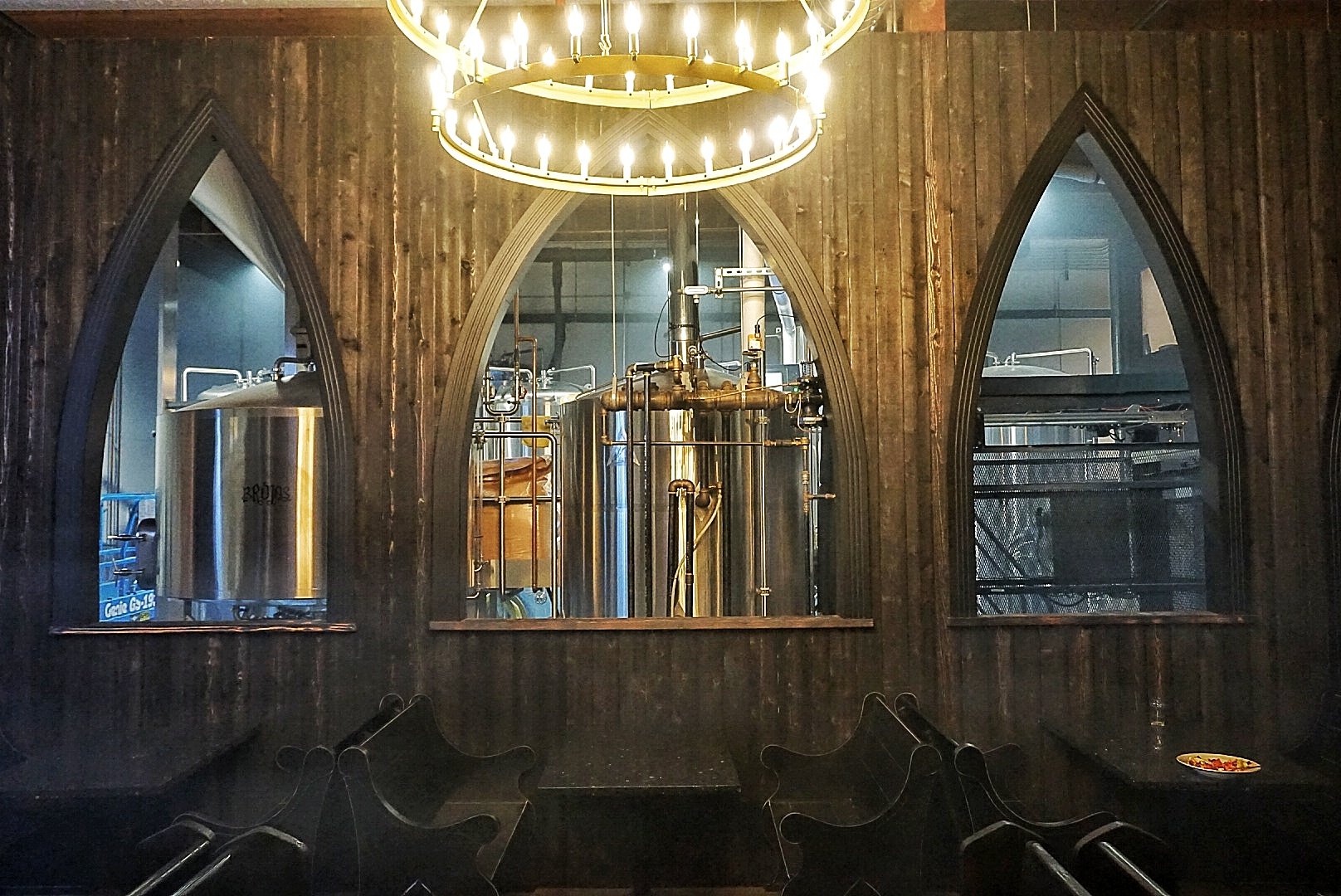In the image, which resembles a painting, there is a spacious room that looks like a beer hall or a factory cafeteria. The foreground features empty tables with pew-like wooden benches, one of which has an unbussed plate with remnants of food. Above these tables, a grand chandelier with circles of bulbs emanates a warm glow. The backdrop is a wooden wall with vertical planks, showcasing three evenly spaced, triangular arched windows. Through these windows, metallic vats or stills are visible, hinting at a brewing operation. The scene is replete with various metallic pipes and lights, adding to the ambiance of a functioning brewery.